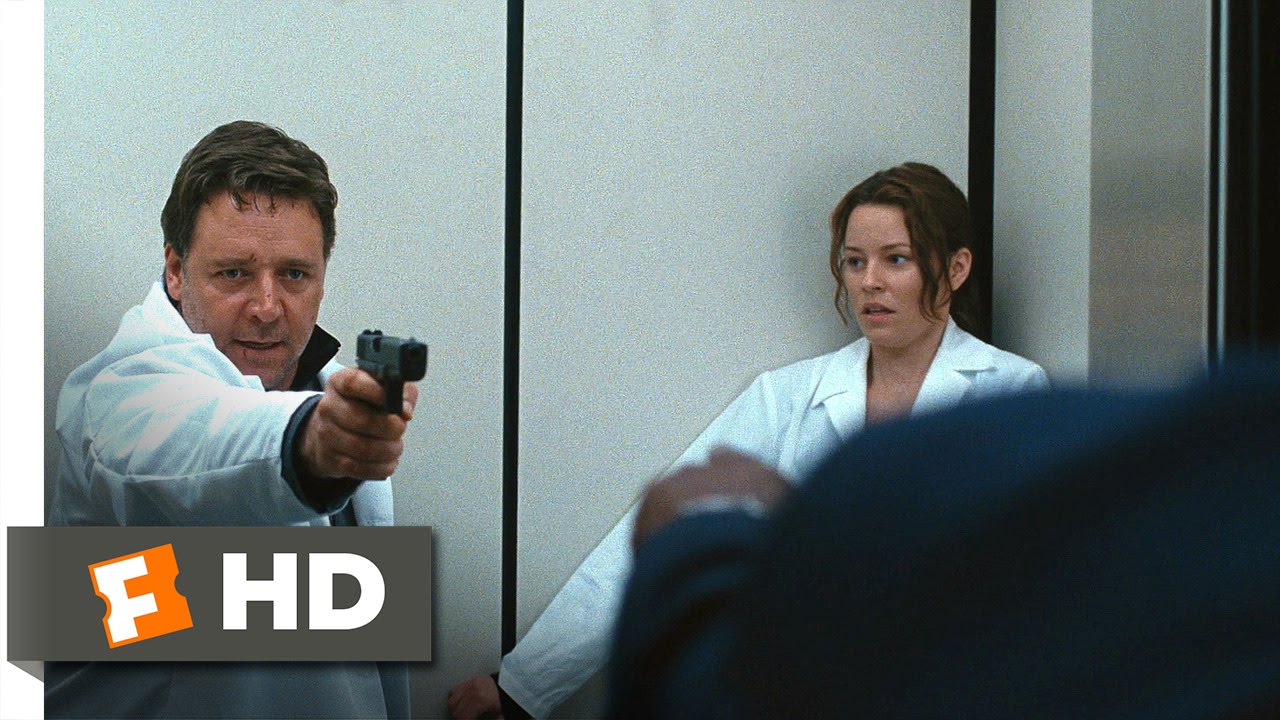In the movie scene, we see a tense moment set in a confined space with white panel walls interspersed with black joints. Russell Crowe, with his short brown hair combed to the right and a concerned expression on his face, is dressed in a white suit jacket over a black suit. He is holding a black handgun, possibly a Glock or a 9mm, pointed towards an unseen person, only part of their shoulder in blue visible from the back. Beside him stands a frightened Elizabeth Hurley, her dark brown hair pulled back with some tresses hanging beside her face. She is clad in a white lab coat and leans against the corner, staring apprehensively at Crowe and the gun. In the background, a woman with brown hair also wearing a white jacket is visible, appearing scared. The image is overlaid with an FHD label on the left, with the 'F' in a white letter inside an orange square and 'HD' in bold white letters on the right.